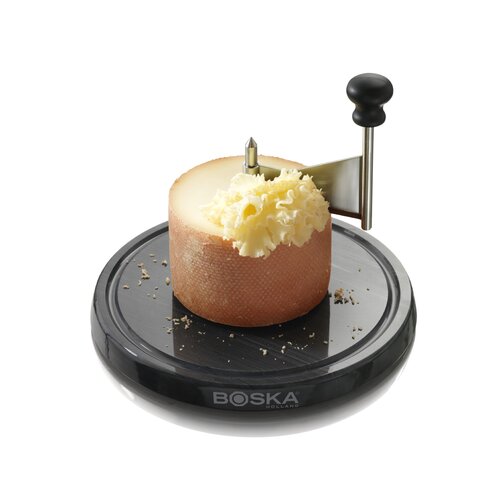The image showcases a modern kitchen appliance designed to shave cheese, likely a cheese curler, set against a completely white background suggesting an online listing. The base of the appliance is a round, black circular platform with an indentation near the outer edge and the brand name "BOSKA" printed in white script. At the center of the base is a wheel of cheese with a darker golden crust and a lighter yellow interior, impaled by a tall, silver metal spike to hold it steady. Extending from this spike is a silver-colored blade with a black handle on the right side, which is used to rotate around the cheese, shaving off stylish, fluffy ruffles. The arrangement is presented to highlight the functionality and aesthetic appeal of the appliance.